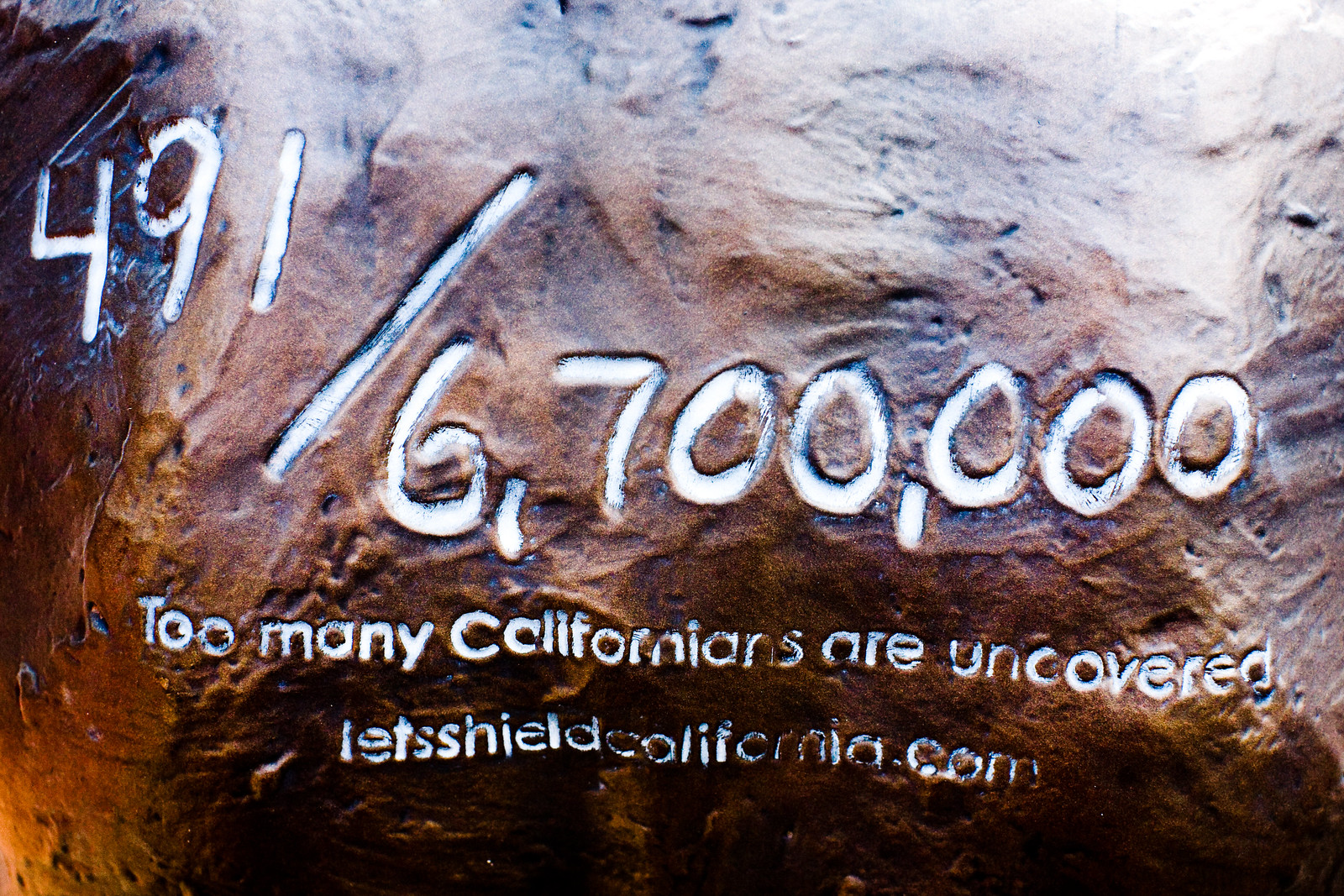The close-up image features a large, somewhat uneven boulder that appears to be a dark brown or bronze color with hints of orange hues, adding to its rugged yet shiny surface. The boulder has text etched into it, painted white for clarity. At the top, the number "491" is prominently displayed, followed by a slash and "6,700,000" below it, occupying the upper part of the image. Beneath this statistic, in smaller, centered text, it reads "Too many Californians are uncovered." The bottom-most part of the image contains the text "letsshieldcalifornia.com," also centered. The latter text takes up the lower third of the image. Dark grooves and markings are visible on the surface of the boulder, adding to its textured appearance.